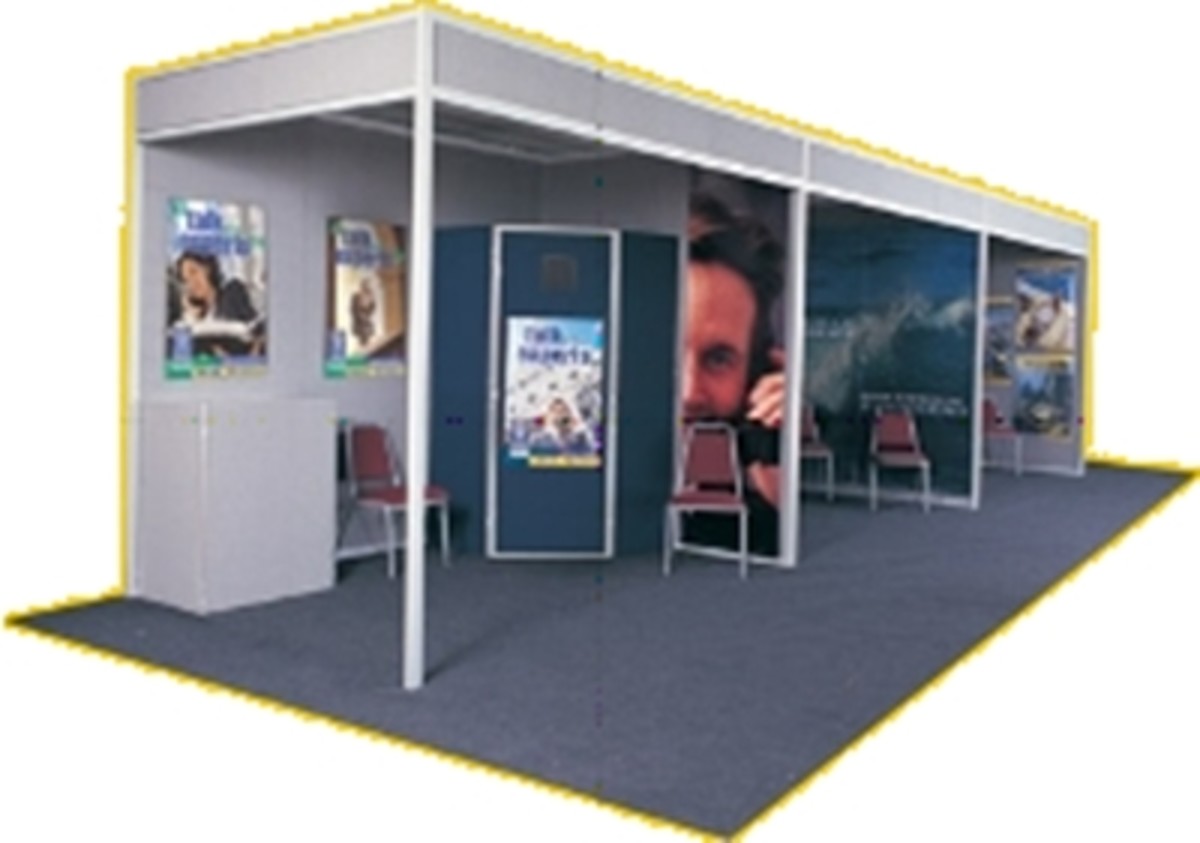The image depicts a meticulously detailed three-dimensional workspace graphic, likely representing an architectural rendering of a modern office or a display area for a trade show or job fair. The space consists of three distinct cubicles, each designed with unique visual elements but unified by a consistent color scheme. The entire setup is framed with a bold yellow border, emphasizing its structured layout.

Each cubicle features a gray carpeted floor and gray walls, accented with white poles for structural support. The walls serve as dividers, creating three separate yet open-ended rooms that are closed at the back and sides but open in the front. Each cubicle is furnished with at least two reddish chairs with silver legs, providing seating within these compact units.

The frontmost cubicle stands out with a blue closet or locker, a silver countertop that could serve as a storage or utility area, and multiple posters decorating the walls. One prominent poster displays an image of a person talking on a phone, suggesting a business or communication theme.

The second cubicle features a serene backdrop of waves with white, unreadable text superimposed, complemented by two red chairs, creating a possibly more relaxed or artistic space.

The third cubicle, though partially visible, showcases various pieces of artwork on the walls, hinting at a more creative or commercial purpose.

Overall, the image captures a versatile, multi-functional environment, accented by thoughtful design elements and color coordination, suitable for professional gatherings, exhibitions, or events.